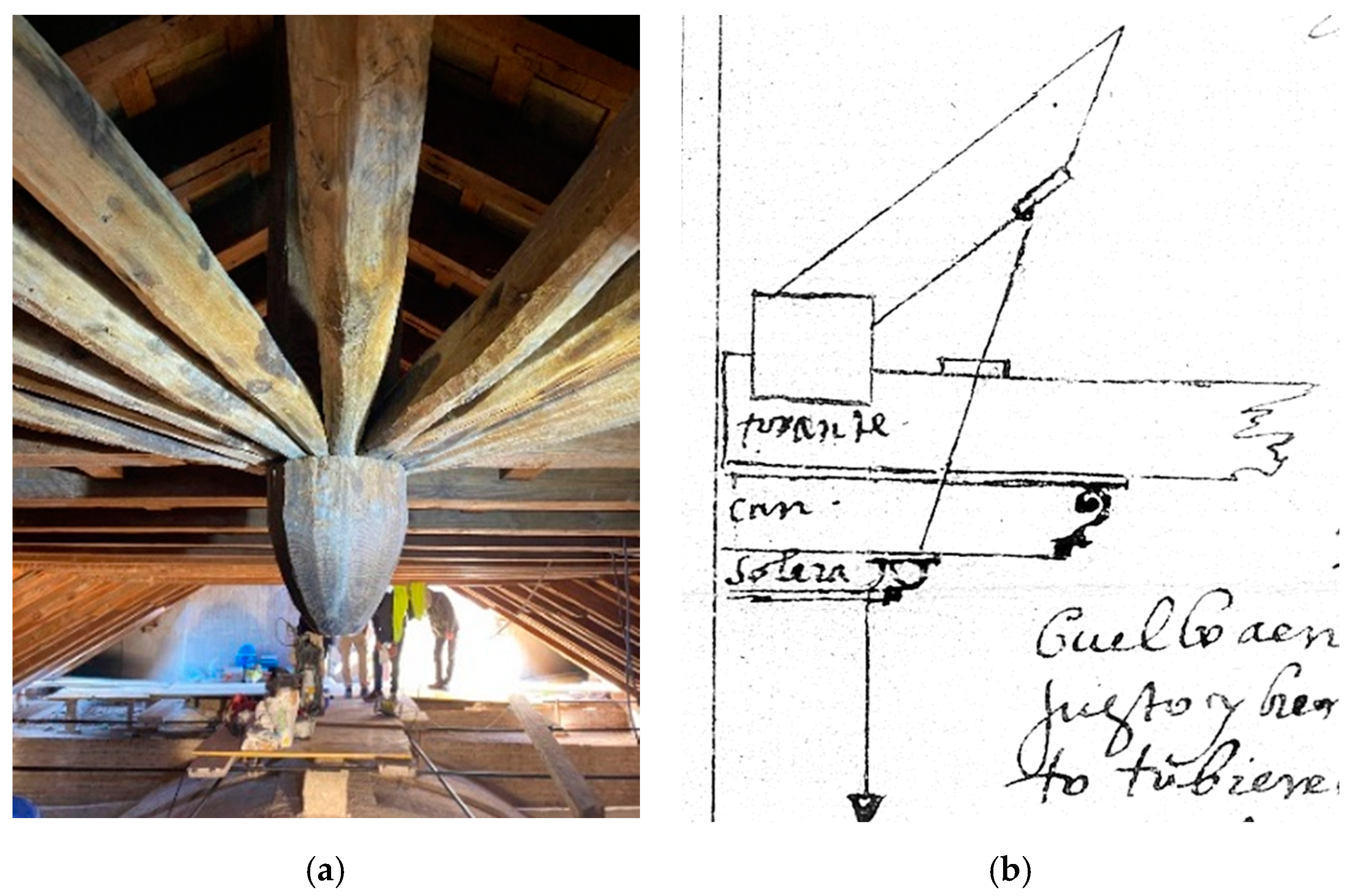This composite image juxtaposes a photograph and an illustration, each labeled with a lowercase "a" and "b," respectively. The photo on the left captures the intricate interior architecture of an old building's attic or roof space, revealing aged, wooden beams converging at a cone-shaped metal joint in the middle. These beams, hand-carved from light golden-tan wood, form a pinwheel design under a triangular, pointed roof. Far below, indistinct human figures suggestive of workers can be faintly discerned. The illustration on the right seems to be a technical sketch related to the photographed structure. It features a diagram with a slanted piece of wood, a string, and a weight-like object, alongside barely legible cursive text and geometric annotations. The diagram potentially represents the structural details or mechanisms within the photographed architecture, implying a connection to mill machinery or similar engineering.